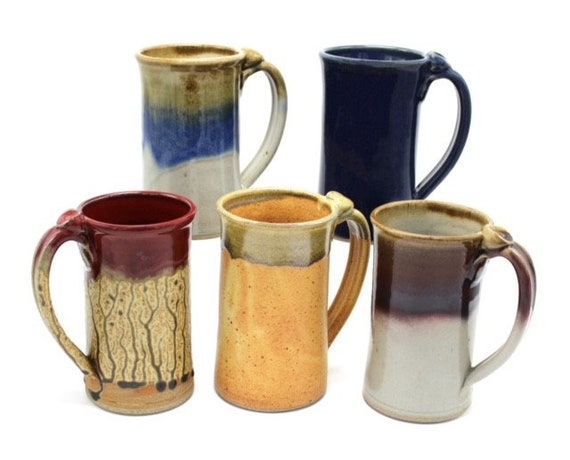This color photograph in landscape orientation features a carefully arranged collection of five tall, handmade ceramic mugs set against a seamless white backdrop, creating an illusion that they are floating. In the back row, the left mug transitions from a white bottom to a light blue middle and a beige top with a right-facing handle. Next to it on the right is a solid navy blue mug, also with its handle oriented to the right. In the foreground, the left mug displays a maroon top with a beige base and intricate brown branch patterns up its side, with the handle on the left. The central mug showcases an orangish-peach hue with a brownish top and right-facing handle. The rightmost mug combines white at the bottom with maroon and gray line patterns on top, its handle facing right. These slender, elongated mugs are noteworthy for their unique, likely handmade designs, distinguishing them from standard mass-produced coffee mugs. The crisp white background emphasizes their artistic craftsmanship, making each piece stand out in vivid detail.